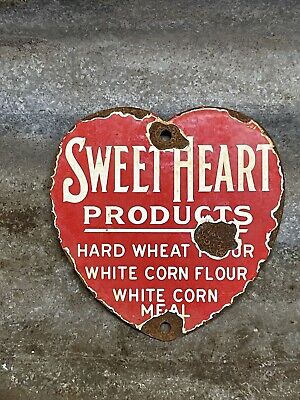The image features a distressed heart-shaped label, with jagged edges and holes at the top and bottom, set against a backdrop that could be either stone, dirt, or a slightly whitewashed wooden surface. The heart-shaped label, which is predominantly red but appears weathered with peeling edges, prominently displays the words "Sweetheart Products" in a large, cursive white font. Below this, in a simpler, smaller white font, are listed "Hard Wheat Flour," "White Corn Flour," and "White Cornmeal." The visual decay and wear suggest the label has been subjected to the elements over time, giving it a rustic and aged appearance.